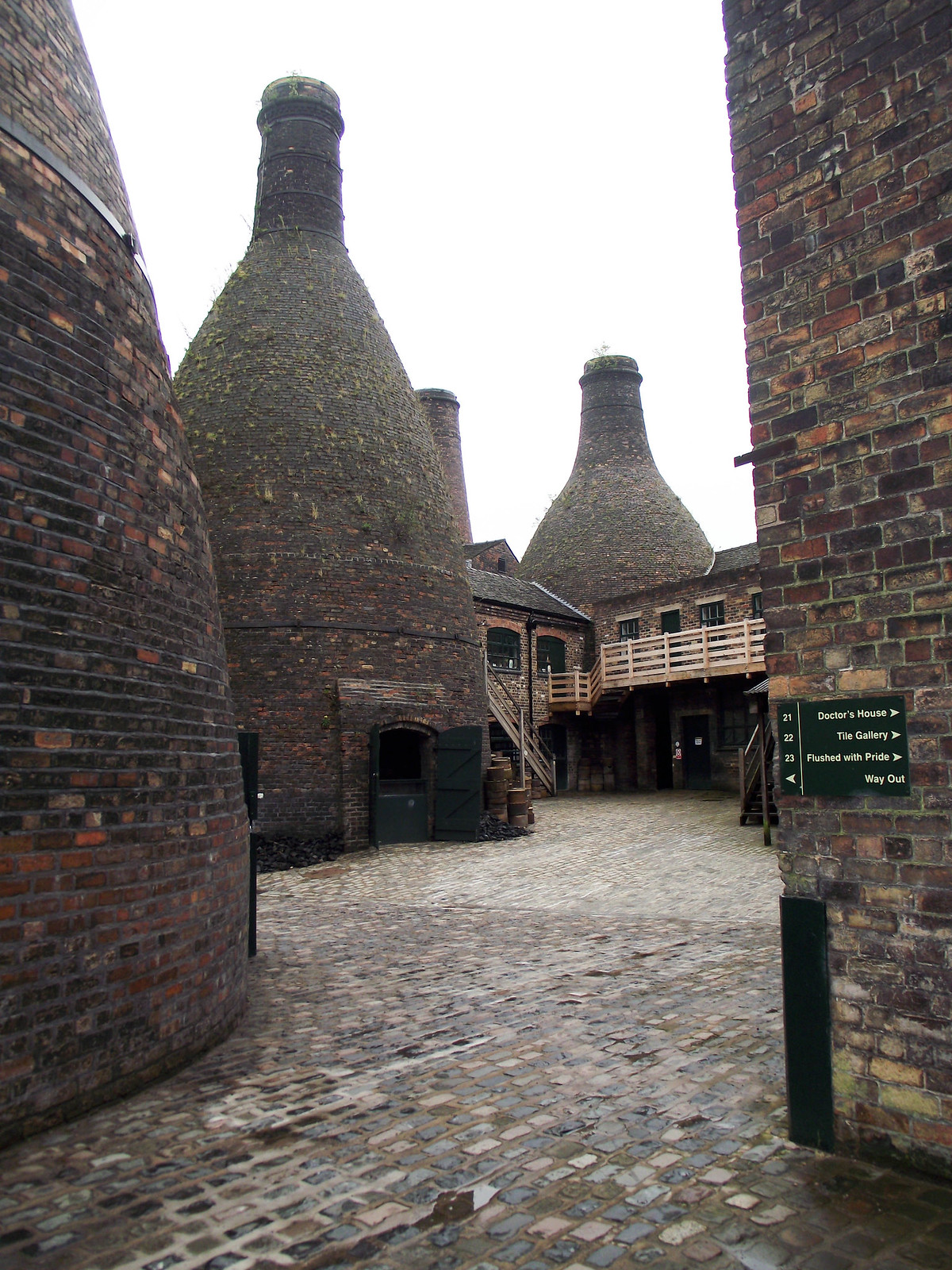This vertically oriented color photograph features the captivating architecture of the Gladstone Pottery Museum, captured on an overcast day. Dominating the foreground are several distinctive, bottle-shaped brick kilns that immediately draw the eye. Constructed from reddish-brown bricks with a weathered texture, these structures taper off to narrow chimneys, reminiscent of antique wine bottles. The scene is set on a cobblestone courtyard, flanked by additional brick buildings and a wooden fence that runs parallel to a low, flat structure.

In the background, a wooden catwalk and steps provide a walkway between different parts of the museum complex, adding to the historical ambiance. A rectangular building with a plaque affixed to its side, featuring names and numbers, suggests directions for visitors. The entire composition of this unique architectural ensemble is unified by the dark, earthy tones of the bricks, contrasting against the bright white, overcast sky, which imparts a moody yet inviting atmosphere.